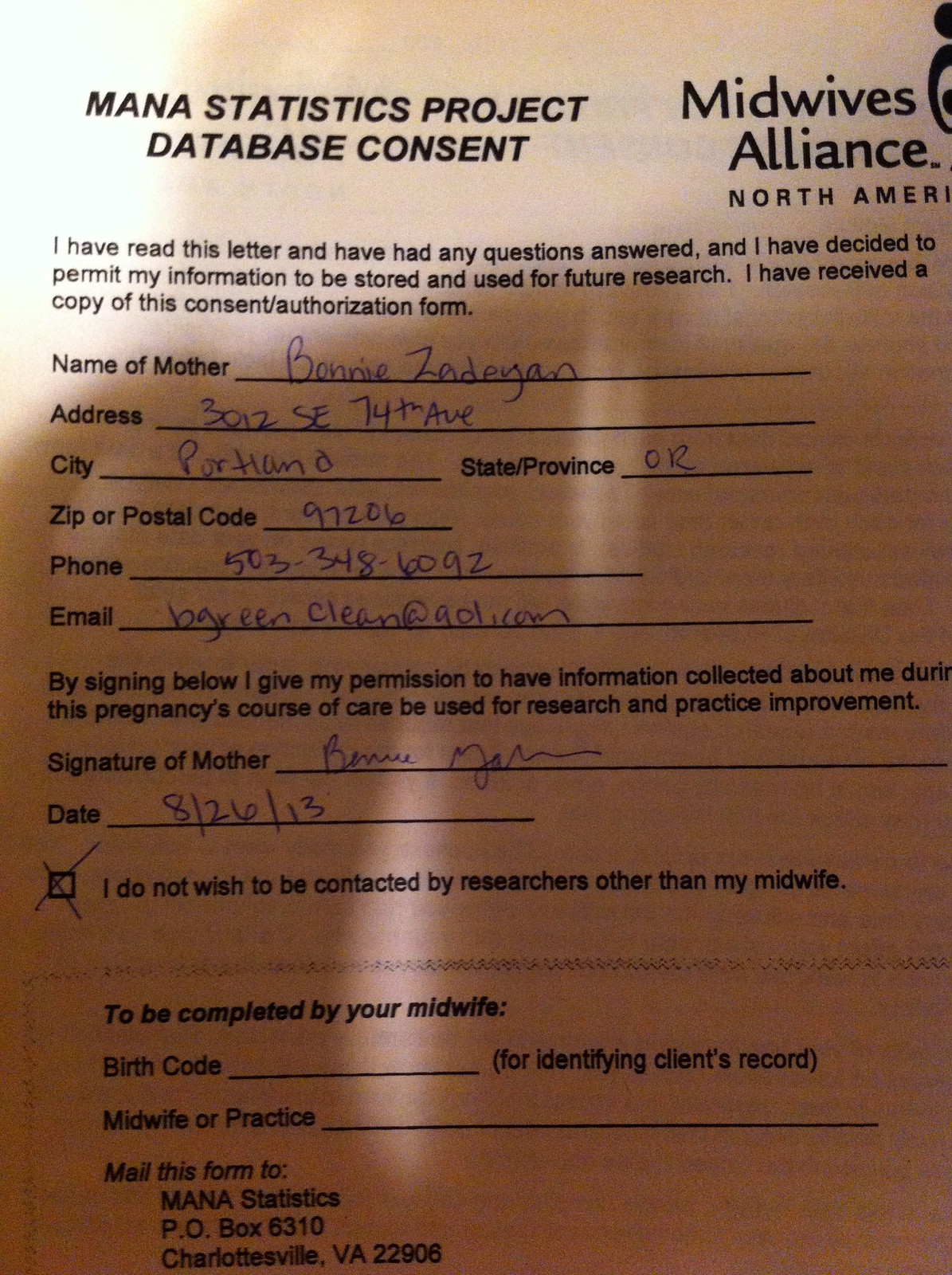This is a brightly-lit photograph of a brown piece of paper exhibiting a significant shadow beneath it. The document, titled "MANA Statistics Project Database Consent," is mainly characterized by its black text. In the upper left corner, the title is clearly stated, while "Midwives Alliance North America" is present on the upper right. This form is a consent authorization for participating mothers to permit the collection and use of their information for future research. 

Key sections of the form include:
- Name of Mother
- Address
- City, State/Province, Zip/Postal Code
- Phone
- Email

There is a checkbox allowing participants to opt-out from being contacted by researchers, except for their midwife. The form includes a detailed consent statement for mothers to acknowledge by signing, indicating their permission for information gathered during their pregnancy care to be used for research and practice improvement. The form ends with fields for the signature of the mother, date, and a section designated for completion by the midwife, including birth codes and identity of the midwife. Lastly, instructions are given to mail the completed form to a specified P.O. box in Charlottesville, VA.